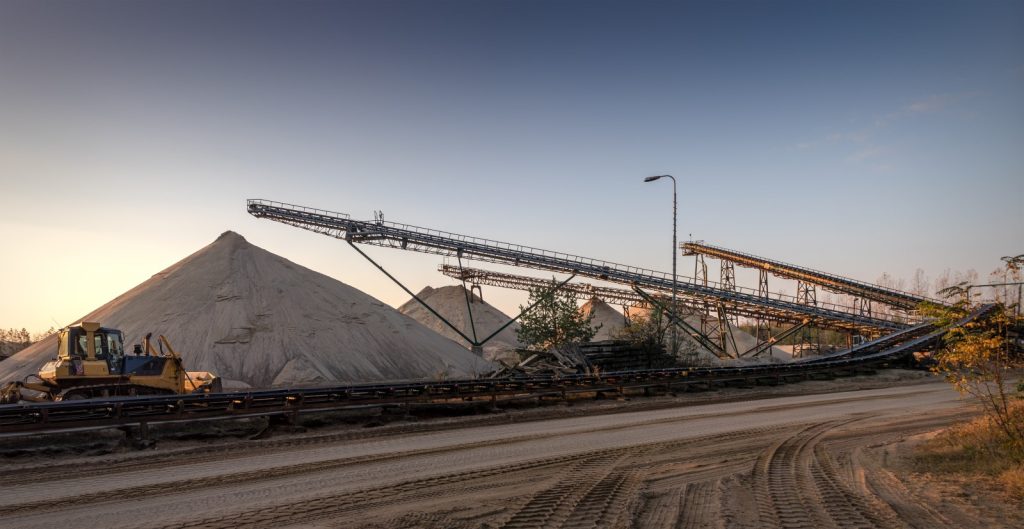The image portrays a daytime outdoor scene of a large construction or mining site, likely a rock quarry. Dominating the lower portion of the rectangular frame is a dirt road under construction, stretching diagonally from the lower left to the middle right, marked with visible tire tracks and accompanied by patches of dirt in the lower right corner. Surrounding the site are small trees, and scattered at various points in the background are tall mounds of tan-colored sand or rock, with more piles visible in the distance.

Central to the scene are three long conveyor belts, extending from the middle right towards the left middle and flanked by a tall street lamp rising above them. These conveyor belts, colored in gold, brown, and gray, are instrumental in transporting the mined material onto the massive sand piles. A caterpillar-type bulldozer or construction vehicle is positioned near the left side of the image, dwarfed by the towering sand mounds, which stand two to three times its height.

The sky, which occupies much of the upper part of the image, is a clear blue, punctuated by a few wispy white clouds. The overall atmosphere of the photo is tranquil, highlighted by the low angle of the sun, suggesting either morning or late afternoon.